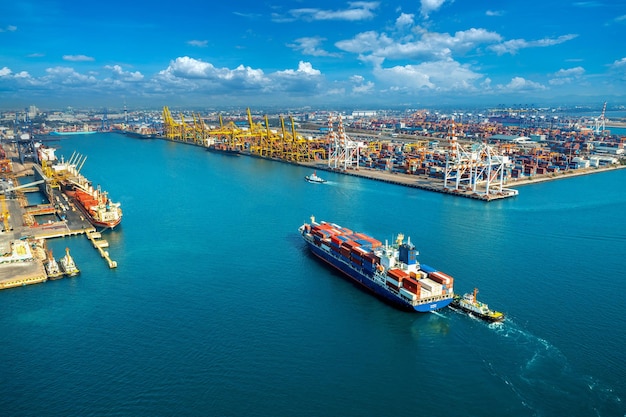This bird's-eye view photograph captures a bustling harbor scene under a vibrant blue sky with scattered clouds, where the azure color of the sky mirrors the calm blue water below. On the right upper half of the image, a floating structure with multiple sections is visible, holding various types of cargo. A channel of matching blue water extends towards the left, with another floating cargo area seen further left in the distance.

Dominating the foreground towards the right, a large container ship laden with red, white, and blue containers is accompanied by a yellow and white tugboat guiding it into the harbor. The ship, characterized by a blue hull and a bridge situated three-quarters towards the stern, appears to be heading towards the bustling harbor to unload its cargo.

The harbor itself is replete with tall yellow and silver metal cranes essential for the loading and unloading process, along with red and white smokestacks towering over the industrial area. Additional ships are anchored nearby, and a network of piers stretches across both sides, lined with buildings painted in various hues of orange, yellow, red, and tan. In the distance, radio towers and other industrial structures dot the landscape, enhancing the view of this active seagoing shipping port.